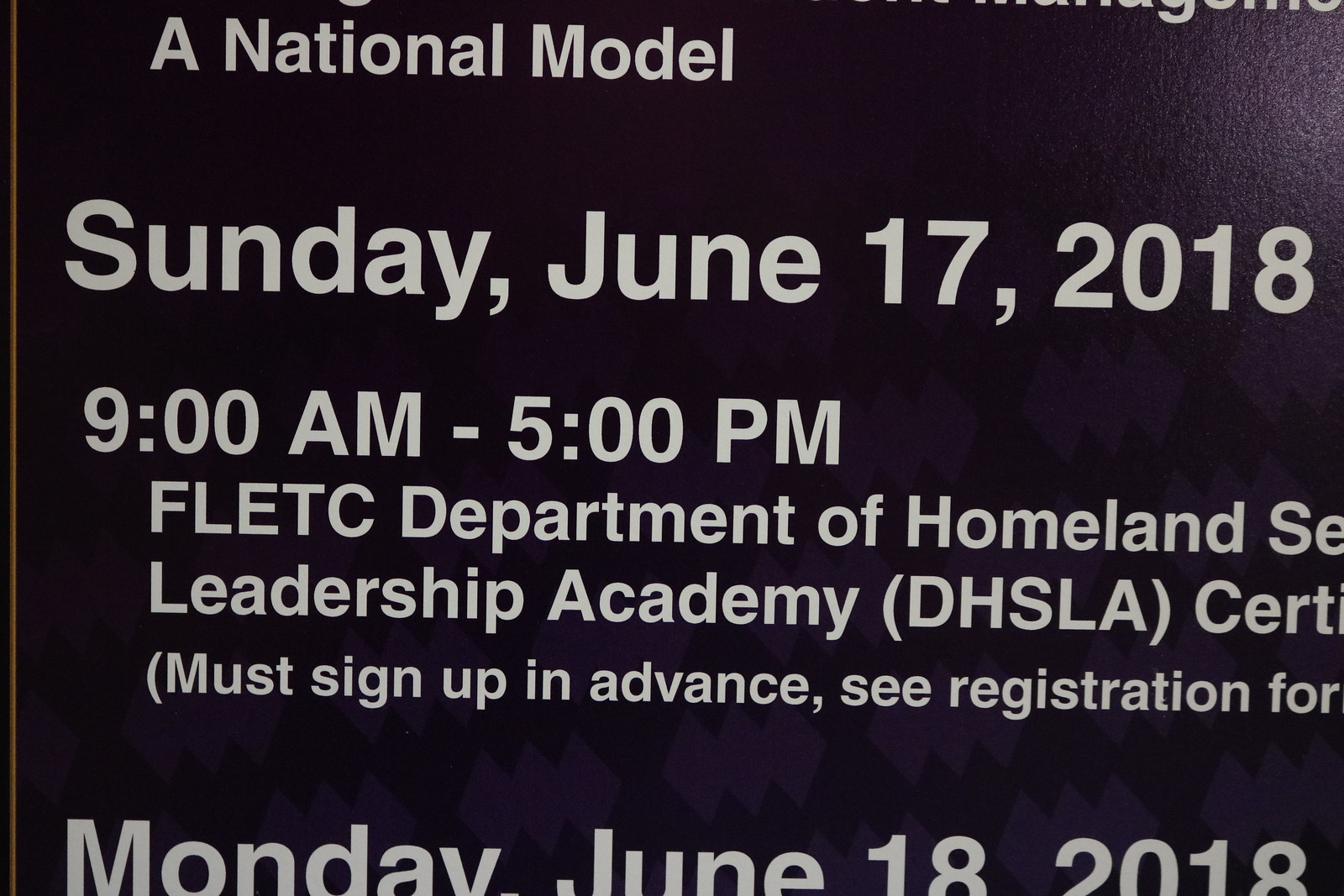The image is a close-up of an informational signboard made of cardstock or cardboard with a black background and multiple lines of white text. Despite some parts being cut off, the readable text details a schedule of events. At the top, in medium-sized letters, it reads, "A National Model." Below that, in larger text, it shows the date "Sunday, June 17, 2018" followed by the time "9 a.m. to 5 p.m." The next lines, in a mix of all caps and regular text, read "FLETC, Department of Homeland SE," likely intended to say "Security." Below that, it lists "Leadership Academy (DHSLA), CERT" with a note in parentheses stating "must sign up in advance, see registration for details." The final line, in large print, reads, "Monday, June 18, 2018," indicating another event.